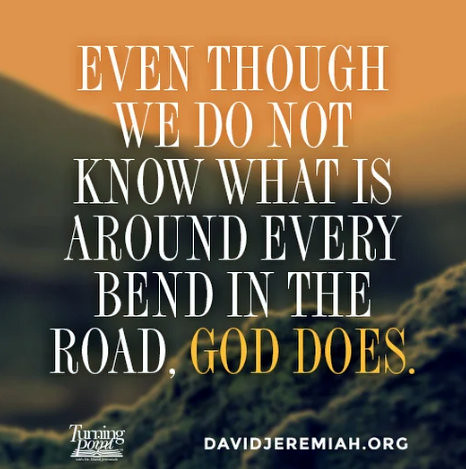The image depicts an inspirational quote imposed on a photograph of a rocky landscape. The foreground features rocks sloping from the bottom left towards the center of the image, leading the eye towards an out-of-focus shadow of a distant mountain. The sky above is an orange hue reminiscent of daytime, though it hints at the warm tones of a sunset. 

Superimposed on this background, the text in white reads, "even though we do not know what is around every bend in the road," followed by "God does" in orange. At the bottom center of the image, white text reads "DavidJeremiah.org," accompanied by a logo to the left that says "Turning Point" in white, next to a graphic of a sideways book. The overall effect is one of tranquil reflection, with the color contrasts and the sloping rocks adding depth to the profound message expressed in the quote.